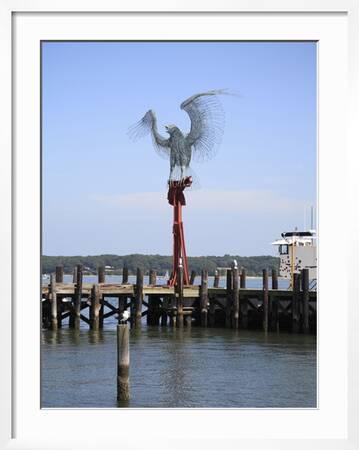The photograph is vertically rectangular and framed in a thin white wooden frame, with a white border inside. The image captures a serene outdoor scene featuring an old wooden dock extending from the left to the right across a calm, brownish-gray body of water with gentle ripples. In the center of the dock stands a prominent statue with a red narrow base; it depicts a large, gray eagle with outstretched wings, appearing to carry something in its claws. To the side, there is a thin, round wooden post emerging from the water, with a bird perched atop it. The upper part of the photograph is dominated by a bright blue sky adorned with thin white layers. The background reveals glimpses of large green trees, enhancing the vibrant and clear setting of this daytime shot.